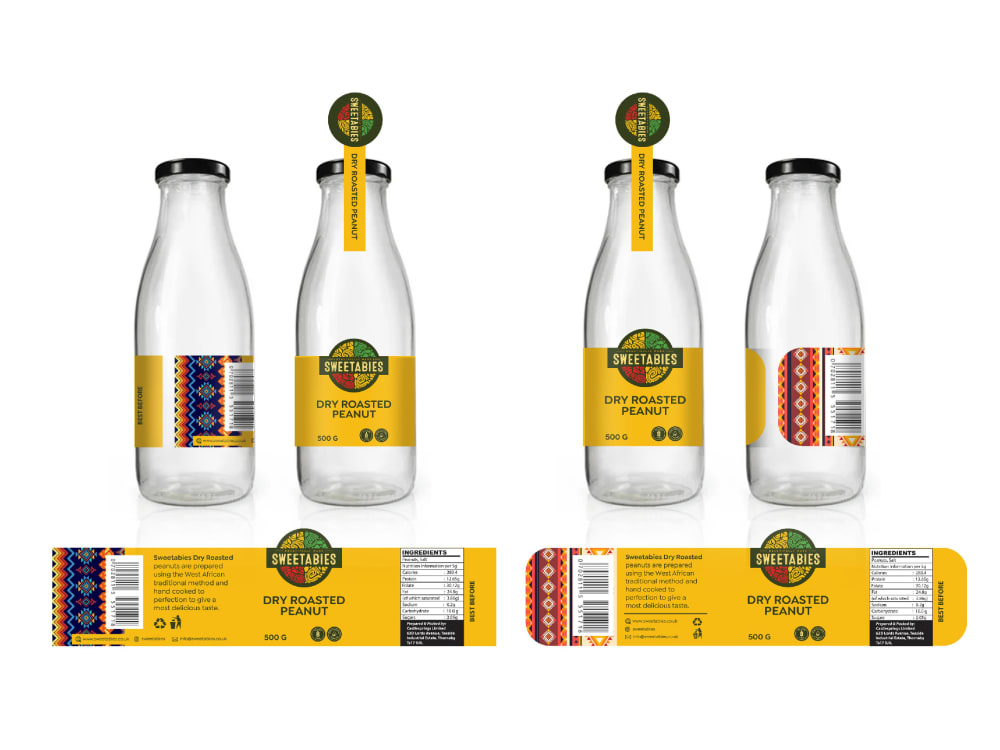The image displays four clear glass jars of peanuts, each with black lids, arranged in pairs. Two jars are shown from the side, displaying a UPC symbol, while the others are viewed from the front, highlighting their labels. These labels are primarily golden-yellow, featuring an olive green rectangle with the brand name "Sweet Habies" in light yellow letters. The product name "Dry Roasted Peanut" is also in olive green. The top of each lid has a paper seal. Below the jars, the image includes two fully rolled-out labels. One label shows a blue and orange pattern, while the other features a pink and turquoise design, suggesting slight variations in design despite the consistent text. The labels detail that "Sweet Habies Dry Roasted Peanuts are prepared using a West African traditional method and hand-cooked to perfection to offer the most delicious taste." The labels also display a recycle symbol, a disposal icon, and the product weight of 500 grams.